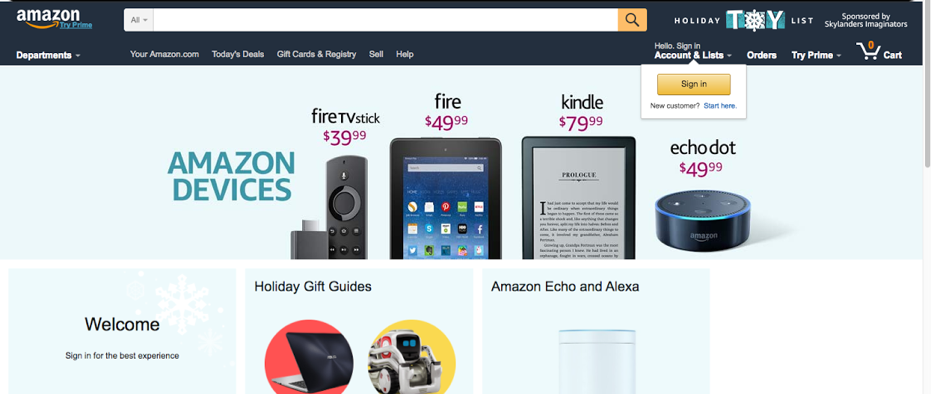Here is a more polished and detailed caption for the image:

The image depicts the landing page of Amazon, characterized by its distinct and structured layout. At the very top, a prominent black navigation bar spans the width of the page, approximately an inch and a half in thickness. Positioned in the top left corner of this bar is the Amazon logo, accompanied by the text "Try Prime" in blue lettering beneath it. Adjacent to the logo is the expansive search bar, followed by a golden search button to its right. 

On the far right of the black bar, there is a mention of the "Holiday Toy List," which is sponsored by "Skylanders Imaginators." Moving slightly downwards within the bar, a secondary menu is visible, listing options such as "Departments," "Your Amazon.com," "Today's Deals," "Gift Cards & Registry," "Sell," and "Help" on the left side. On the right side, it displays options for user interaction including "Hello, Sign In," "Account & Lists," "Orders," and another invitation to "Try Prime," as well as a shopping cart icon indicating zero items. 

Beneath the black bar, there is a section tinted in shades of light blue, featuring three distinct light blue squares. The top segment promotes Amazon devices, highlighting products like the Fire Stick, Fire Tablet, Kindle, and Echo Dot. Below, the three squares detail various promotions: "Welcome," "Holiday Gift Guides," and "Amazon Echo & Alexa." This concise yet descriptive layout captures the essence of the Amazon landing page, offering a clear navigation and a wide array of shopping options.